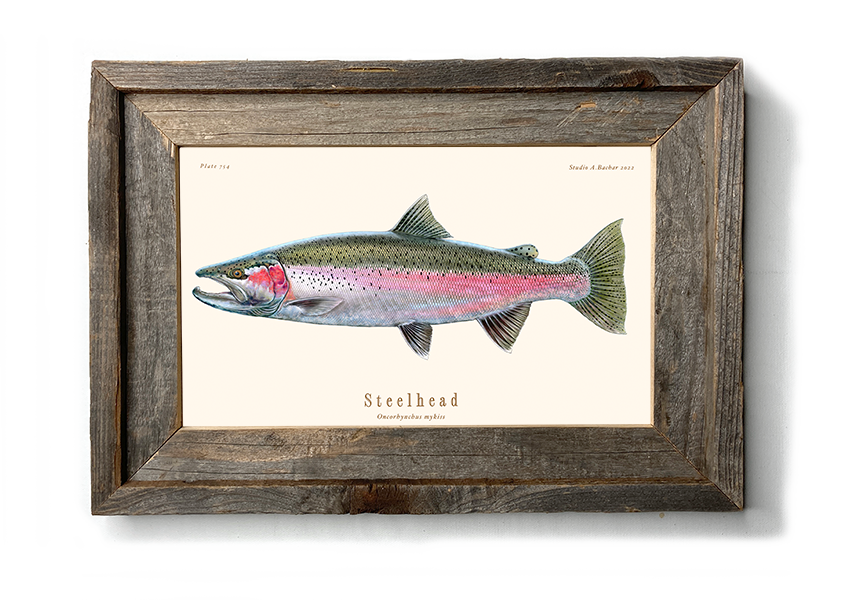This photograph depicts a framed illustration of a steelhead fish. The fish, identified by the text "steelhead" beneath the drawing, is depicted with a predominantly green top, a pink streak running lengthwise along its midsection, and a silvery white belly. The illustration displays intricate details with black dots scattered across its scales, red spots near the gills, and a curvaceous mouth that appears somewhat menacing. The fins are also tinged with olive green, adding to the vibrant palette of the image.

The frame, crafted from a thick, aged medium-colored wood—possibly old driftwood—encloses the picture, consuming about 20% of the photograph's periphery. This rustic frame imbues the image with a vintage charm, suitable for a hunting or fishing cabin. In the top corners of the illustration, there is barely legible text which might read "Studio A Becker 2022" and possibly a plate number "764."

The steelhead fish's scientific name is included under the type identifier, although it appears somewhat indistinct and might read "Oncorhynchus mykiss." The image, set against a white background, is a detailed and lifelike representation of this aquatic species, extending across the entirety of the frame.